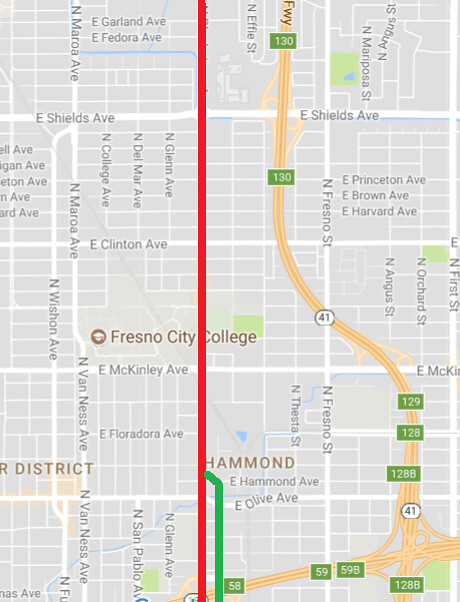This is a detailed screenshot of a map, likely viewed on someone's phone. The map features multiple street views and labels from top to bottom. A prominent straight red line runs vertically down the center of the screenshot, intersected by a green line and further accented with an orange, squiggly road marking in the bottom right corner. The map highlights various crisscrossing roads, each marked with street numbers. Some numbers are encased in white circles with black borders, while others are set against a green background with white text.

Key landmarks include Fresno City College and the Hammond District, with a multitude of street names crisscrossing from right to left. The overall background of the map is predominantly gray, with side streets marked by white blocks. Potential parks are depicted in shades of blue and light green.